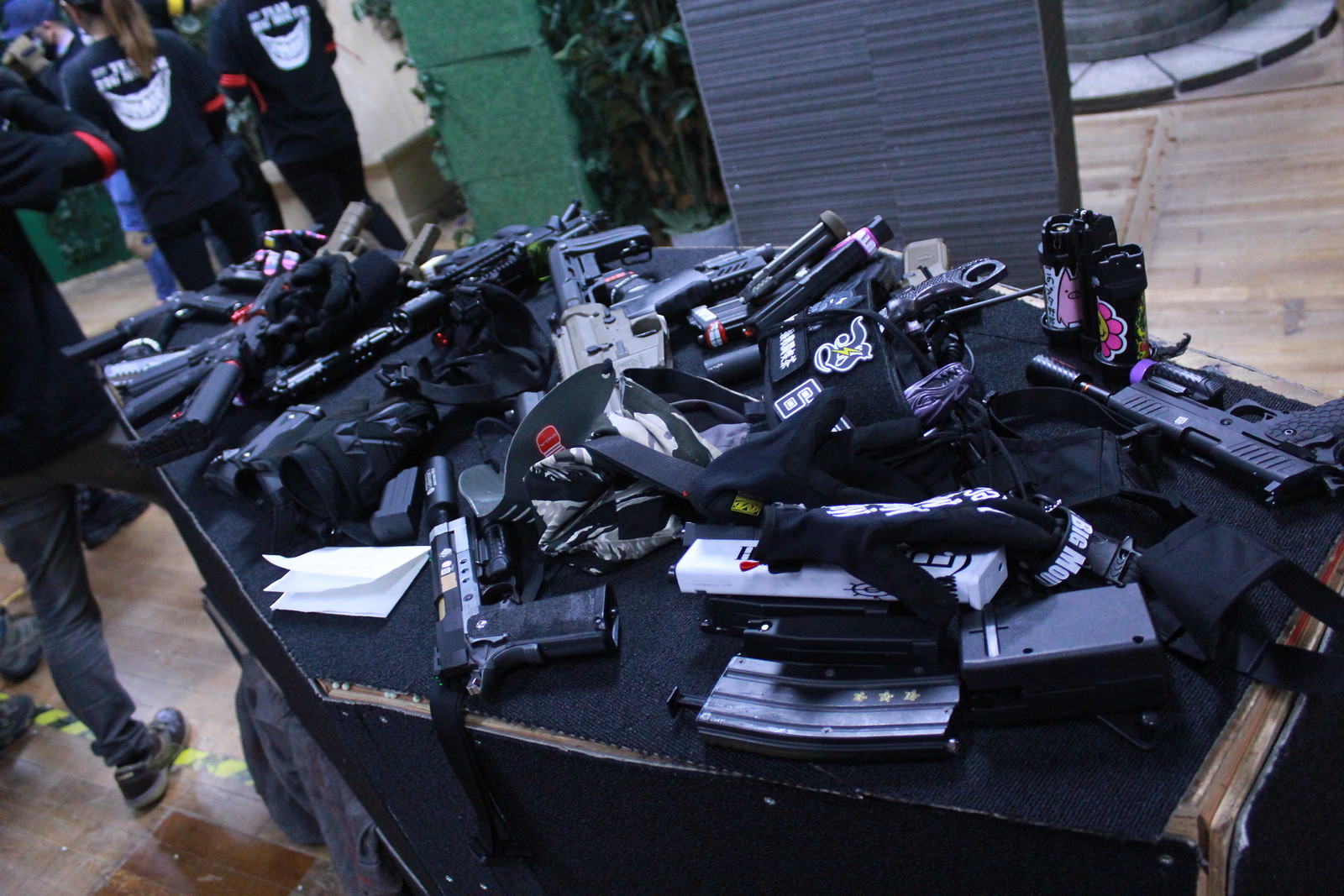The image showcases a cluttered scene of various firearms and magazines scattered across a black fabric-covered table, situated in a room with a brown, particle board floor. The firearms, primarily black and gray handguns, include some with silencers and a machine gun with a brown body and black parts. Among the pile are miscellaneous items such as black gloves, holster straps, folded white paper, and two smoke bombs with pink designs. In the background, three individuals are visible: two women in black t-shirts with a white graphic and red designs on the sleeves. The environment features green vertical displays and walls, contributing to the disorganized appearance of the setting.